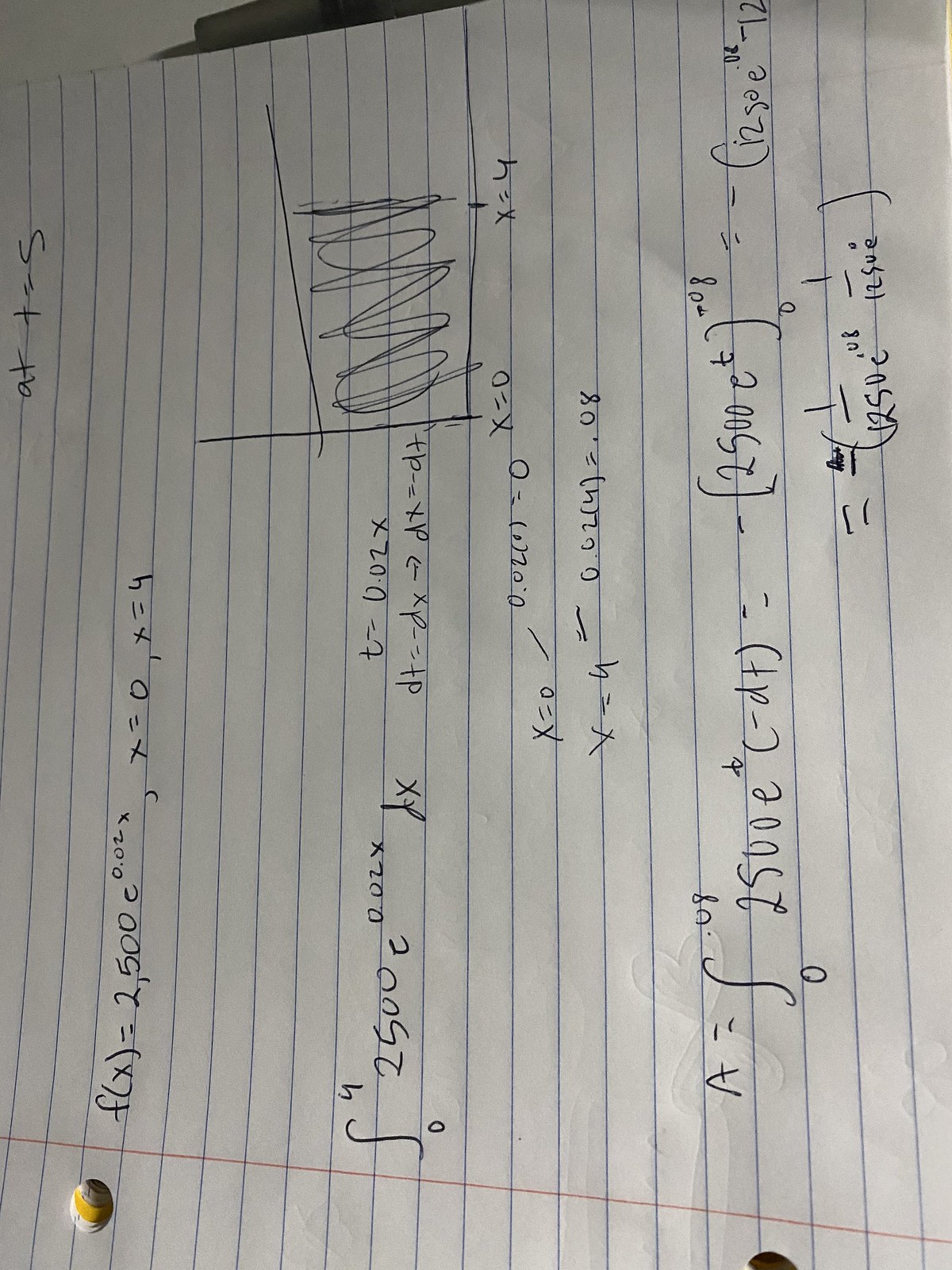This image showcases a piece of white notebook paper, oriented sideways, necessitating a tilt of the head to read its contents. The notebook paper has distinctive blue horizontal lines interspersed with a vertical red margin line on the left, aligned with the three punch holes meant for binder insertion. The page is densely populated with various equations and mathematical notation. Among these, notable inscriptions include "LFLX = 2,500 C," "X = 0," "X = 4," and recurring patterns like "T = UO2" and "DT = DX = DX = DT," with "X = 0" reappearing next to "X = 9." The handwritten text is accompanied by sporadic scribbles, enhancing the impression of a working draft or study notes.